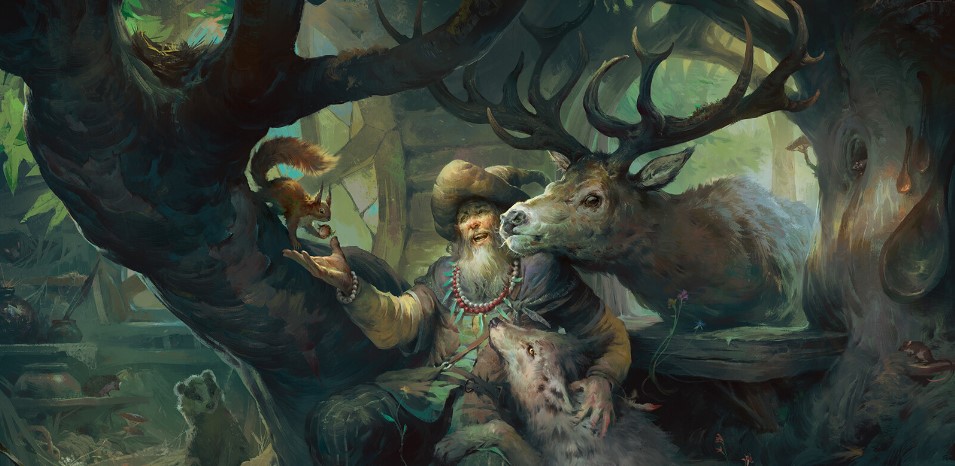This detailed illustration, reminiscent of a storybook or cartoon, portrays a serene, dark-themed scene dominated by earthy colors—predominantly browns, reds, blues, yellows, and shadows. At the center, a bearded man, who seems wizard-like, complete with a tan, traditional wizard hat, sits by a large tree. He is dressed in layered clothing: a blue short-sleeved shirt over a long-sleeved yellow one, adorned with beaded necklaces—one white and another red with green feathers.

Surrounding the man are various woodland creatures, emphasizing his harmonious relationship with nature. To his right, a majestic reindeer with sprawling antlers peers close to his face, while a wolf lies beside him, receiving a gentle pet. A brown squirrel perched on the tree offers him a nut, seemingly in a friendly exchange. In the background near the lower left corner, a small badger looks on curiously from a distance. The setting appears to be either just outside or inside a building, with visible light through a window suggesting daylight. The absence of text focuses attention on the lively interaction between the man and his animal friends, highlighting a peaceful coexistence in this enchanting forest scene.